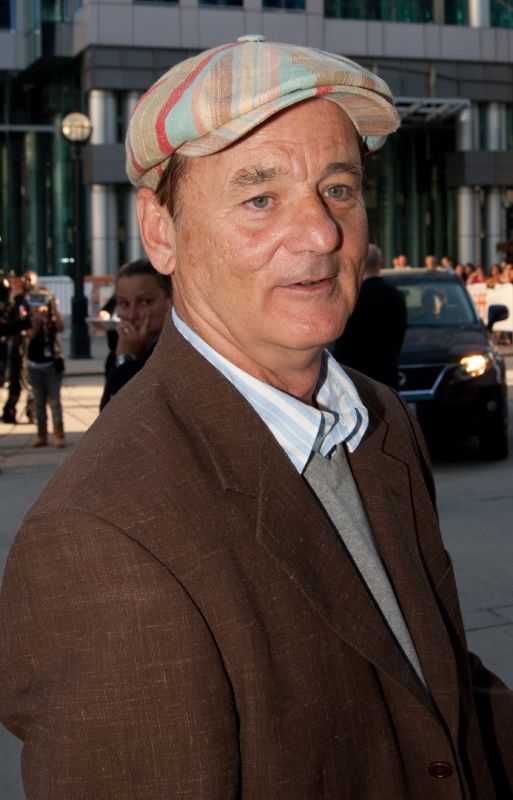The image depicts the actor Bill Murray standing on a city street, facing slightly to the right of the camera, visible from the chest up. He has dark brown hair and blue eyes. He is wearing a unique, multicolored taxi-style cap with red, blue, brown, and beige stripes, featuring a button on top and a brim. His outfit consists of a gray v-neck sweater layered over a blue and white striped collared shirt, and a brown jacket worn open over these layers. In the background, a streetscape is visible with pedestrians walking, a black SUV with its headlights on to his right, and a large gray office building with silver columns. The colors in the image include black, brown, blue, white, gray, red, light blue, light green, tan, and beige, contributing to the vibrant city scene. Bill Murray's presence is prominent, making him the main focus of the photograph.